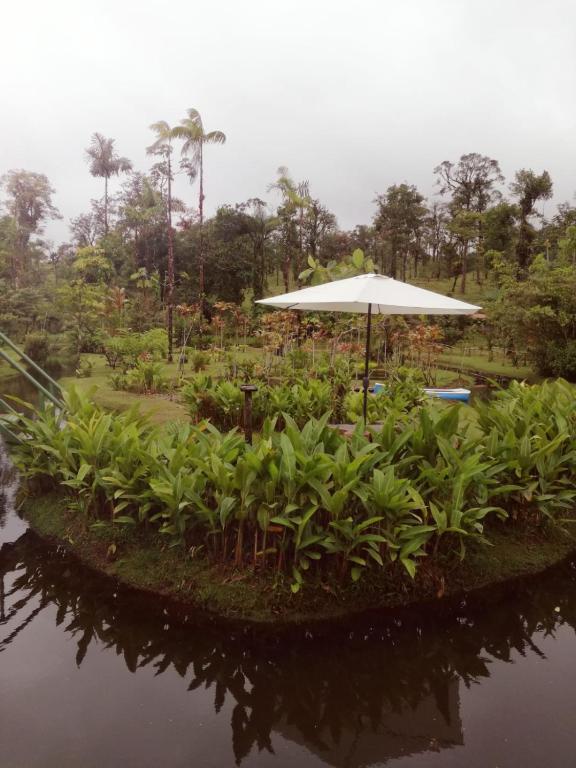This photograph captures a serene, tropical outdoor setting. In the foreground, there is a river or creek that curves around a bend, reflecting the lush green shrubs on its banks. These shrubs include tall, fern-like plants and banana trees. Just beyond the water, there's an island or peninsula adorned with a white sun umbrella standing above a table, creating a tranquil resting spot surrounded by additional greenery and grass. In the background, a small white-and-teal rowboat is docked along the water's edge. The scene is framed by tall, verdant trees and palm trees, with a grayish-white sky overhead, suggesting a recent rain. The entire landscape exudes a tranquil, tropical ambiance.